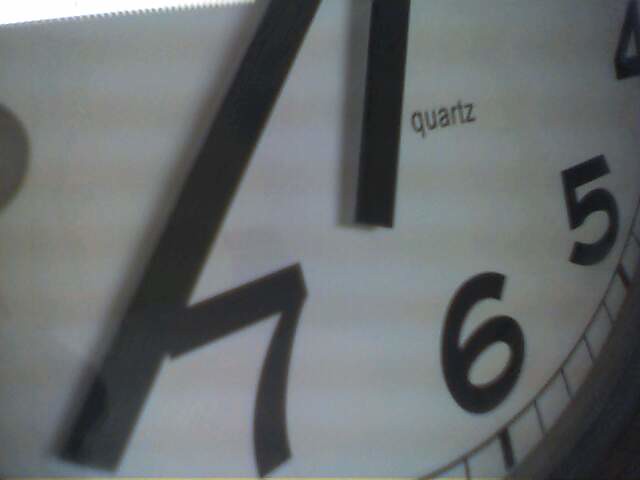In this highly detailed close-up image of a clock's lower section, we see a zoomed-in view focusing on the bottom part of the clock face. On the far right, the image shows a cut-off portion of the number "4" in black. Adjacent to this partial numeral, the numbers "5" and "6" are prominently displayed at the bottom, with the number "7" positioned directly in front. To the left, a faint shadow indicates where the "8" would be.

The word "Quartz" is inscribed in small, black text. Positioned above this text are the two clock hands, both rectangular in shape and black in color. The hour hand is situated between the "7" and the shadow of the "8," while the minute hand extends just beyond the "7." The bottom of the clock face features a pattern of very thin lines running vertically along the outer edge. In the lower right-hand corner, part of the clock’s dark gray outer frame is visible, providing a contrast to the predominantly black and white elements of the clock face.